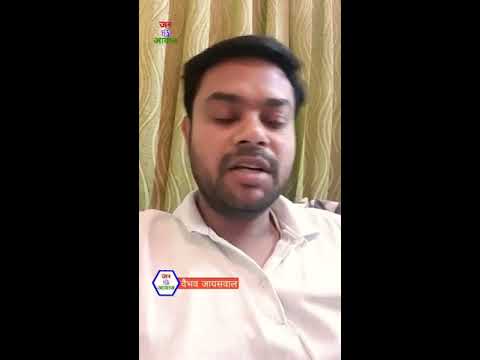In this image, which appears to be a screenshot from a video, a man in his late 20s or early 30s is the central focus. He has a close-cut beard and dark mustache, and his short dark hair complements his fair, caramel complexion. The man is wearing an off-white, buttoned-up polo shirt with no decorations and is positioned centrally in the frame. He looks like he might be speaking, with his eyes seemingly closed and his mouth slightly open. 

Behind him, gold curtains are drawn, adding a warm backdrop to the scene. The image quality is poor, making it difficult to decipher the text in the top left corner and the lower left corner, both of which are in an Asian script, possibly Indian. The text in the top left appears to be green and red, while the lower left contains a red banner with white text and a yellow or white pentagon with a blue outline. The entire photograph is framed with two thick black bands on the left and right, suggesting it was captured on a cell phone.